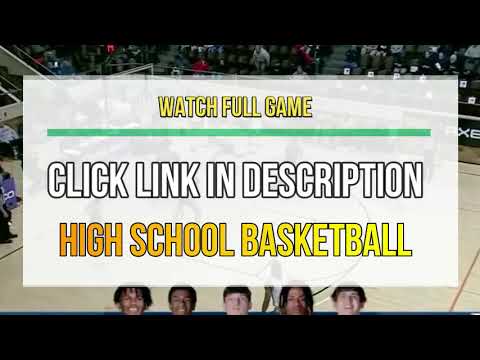This letterboxed photograph, shaped like a high-definition television screen with black bands at the top and bottom, showcases a high school basketball scene. Centered in the image is a semi-transparent rectangular white text box. The text box prominently displays the phrase "WATCH FULL GAME" in bold yellow text, underlined by a green line. Below this, in all caps white text with a black outline, it reads "CLICK LINK IN DESCRIPTION." The phrase "HIGH SCHOOL BASKETBALL," also in bold yellow text with a black outline, appears at the bottom of the text box. Behind the text box, the background reveals a basketball court and stands. The heads of five players are visible at the bottom of the court, emphasizing the game's setting and atmosphere.